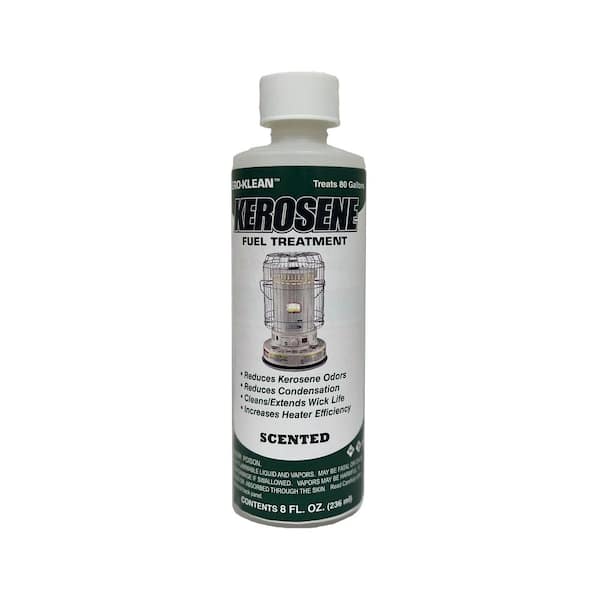This is a detailed photo of a white cylindrical bottle with a twist-off cap, labeled for kerosene fuel treatment. The label is primarily white with green accents at the top and bottom. Prominently displayed at the top in large black capital letters is the word "KEROSENE," followed by "FUEL TREATMENT." The label features an image of a silver steel kerosene lamp, which appears to be suitable for tabletop use. The bottle advertises several key benefits including reducing kerosene odors, condensation, and extending wick life, while also increasing heater efficiency. Additionally, it notes the liquid is scented. Essential product details include the volume of the contents, 8 fluid ounces (236 milliliters), and a precautionary note at the bottom in white capital letters indicating that vapors may be harmful.